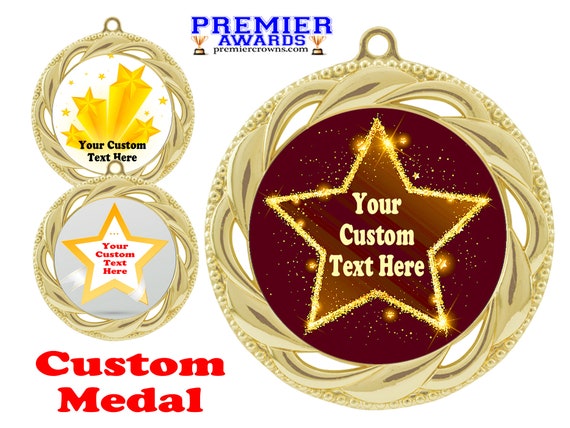The image is an advertisement for medals from Premier Awards, featuring their website, premierecrowns.com, prominently at the top. Centrally, there is a large round medal with a star at its center, inscribed with "your custom text here." This outer gold-lined circle has intricate detailing, including tiny circles with dots and swirling gold patterns with gray lines. The star in the middle is gold with gold flakes around it, set against an amber background with additional gold stars shining.

On the left side of the image, two smaller medals are displayed. The upper one features yellow shooting stars on a white background, with "your custom text here" written in black. Below it, another medal with a white interior and a blue background highlights a large yellow star and "your custom text here" in red. Both smaller medals are also framed in gold.

At the bottom of the image, bold red lettering says “custom medal,” tying the advertisement elements together, pointing out the customizable nature of these ornate and detailed awards.